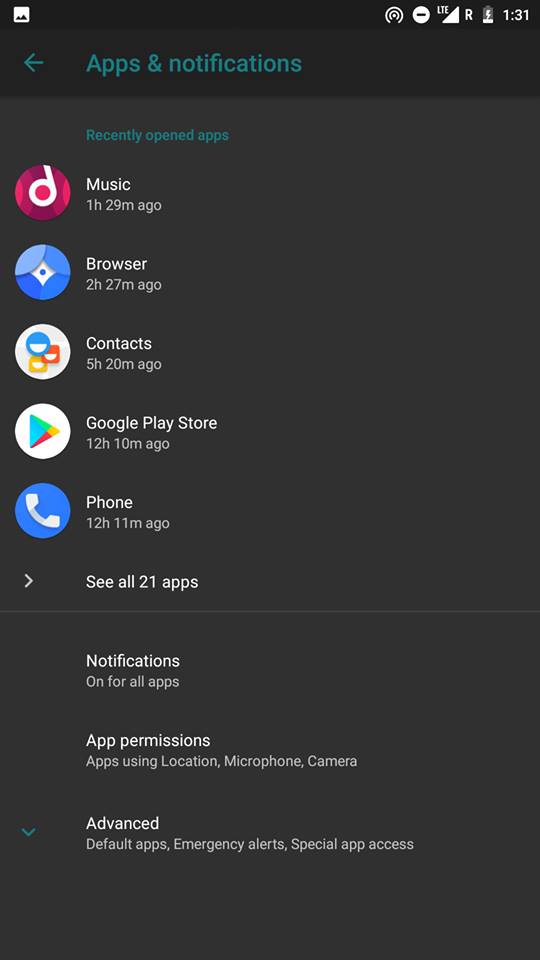The image is a rectangular screenshot taken from a smartphone in portrait mode, with the longer side of the rectangle oriented vertically. The entire background is a dark gray or black. At the top, there's a black banner featuring various status icons. On the top left, there's a small white box containing a mountainscape icon, suggesting this might be an image or photo app icon. Moving to the right, there's an icon of concentric circles with an opening at the bottom, possibly indicating a notification or location service. 

Further to the right, there's a white circle with a horizontal white line inside it, displaying the label "LTE" and a signal strength of four bars. Next to that, there's an "R" symbol, which could stand for roaming, followed by a battery icon indicating that the phone is charging. The current time shown is 1:31.

Below this banner, the section is labeled "Apps and Notifications," with a left-pointing arrow beside it, likely for navigating back. The subsection titled "Recently Opened Apps" lists several apps that have been accessed recently, including Music, Browser, Contacts, Google Play Store, Phone, and C21 among a total of 21 recently opened apps.

Further down, there's an icon labeled "Notifications," followed by categories such as "App Permissions" and "Advanced." Under the Advanced section, additional options are listed, including "Default Apps," "Emergency Alerts," and "Special App Access."